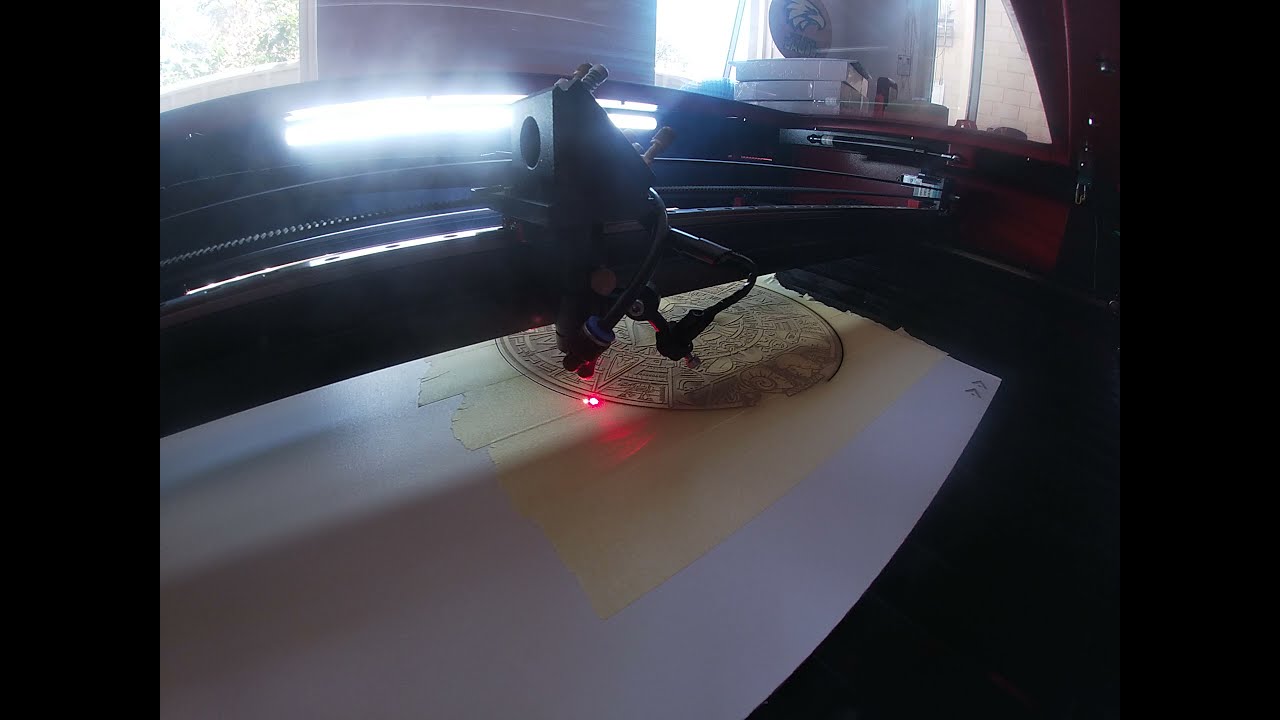The image portrays an indoor setting, likely a home or office, featuring a large 2D printer or laser etching tool positioned prominently in the center. The equipment is actively using a red laser to intricately carve a circular pattern into a white fabric or board-like material. The scene is well-lit with a particularly bright light illuminating the printer space, enhancing visibility of the detailed work being done by the laser. Surrounding the central printer, the background showcases multiple windows indicating daytime, along with various books and boxes scattered around, suggestive of an arts and crafts room. The array of colors visible includes black, white, yellow, red, tan, gray, orange, blue, and green, adding to the vibrant atmosphere of the workspace.